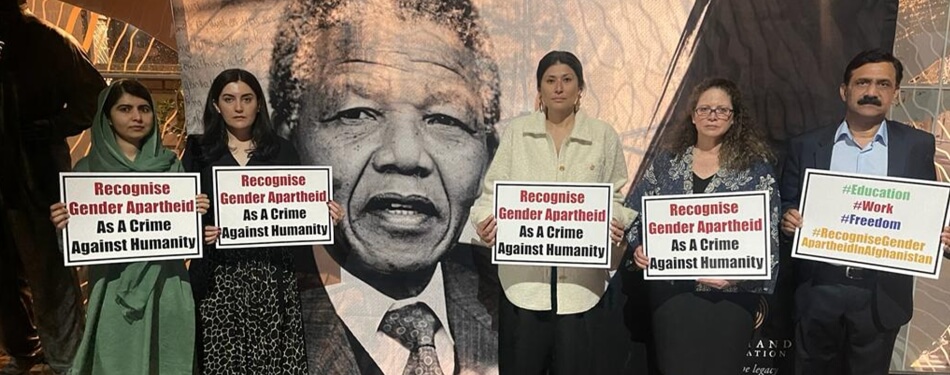In this photograph, a group of five activists stands in front of a mural depicting Nelson Mandela, the iconic anti-apartheid leader and former President of South Africa. These activists include four women and one man, each holding protest signs. The women, who appear to be in their 30s and of diverse races, hold identical signs stating "Recognize Gender Apartheid as a Crime Against Humanity," with the top half of the text in red and the bottom half in black. The man, distinguished by his mustache, holds a sign featuring hashtags that highlight "Education," "Work," and "Freedom," along with a call to "Recognize Gender Apartheid in Afghanistan." This scene suggests a unified global movement against gender apartheid, possibly linked to current events in Afghanistan.